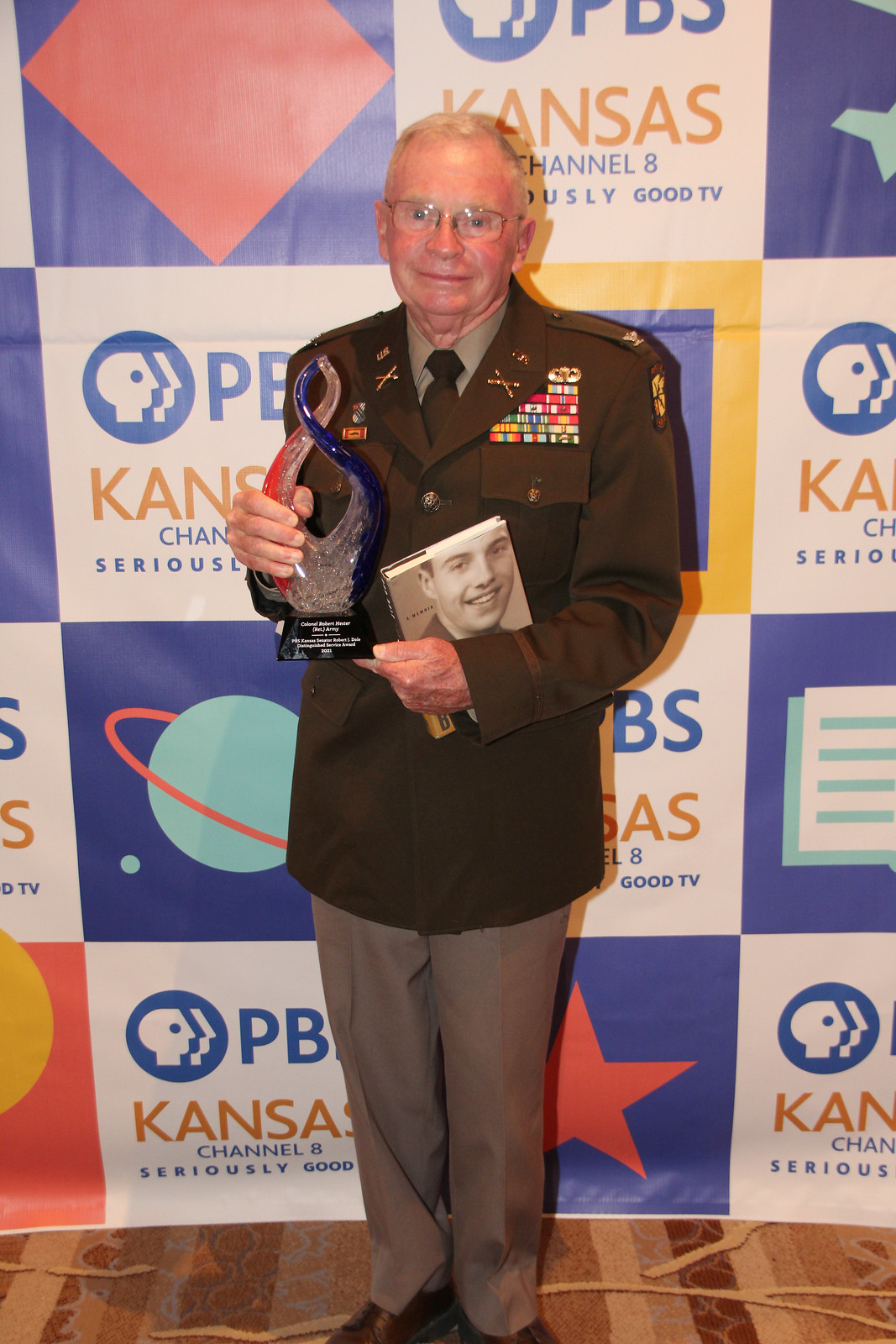This detailed photograph captures an elderly man with white hair and glasses, dressed in a brown military uniform adorned with numerous colorful pins and ribbons. He stands on carpeting in front of a backdrop consisting of blue and white checkered squares, with the white squares prominently featuring the PBS Kansas Channel 8 logo and the blue squares potentially displaying celestial designs. The man has notably pink skin and holds a book, with his right arm supporting it beneath his left forearm. The back cover of the book features a man's face, possibly his own. In his left hand, he holds a distinctive glass award, composed of clear, blue, and red elements, with a swirling white and blue design on a black plaque inscribed with white text. He completes his appearance with gray slacks and black shoes, set against a backdrop indicating "PBS Kansas, Channel 8, Seriously Good TV." The image appears to be taken during an award ceremony, encapsulating his achievements and formal recognition.